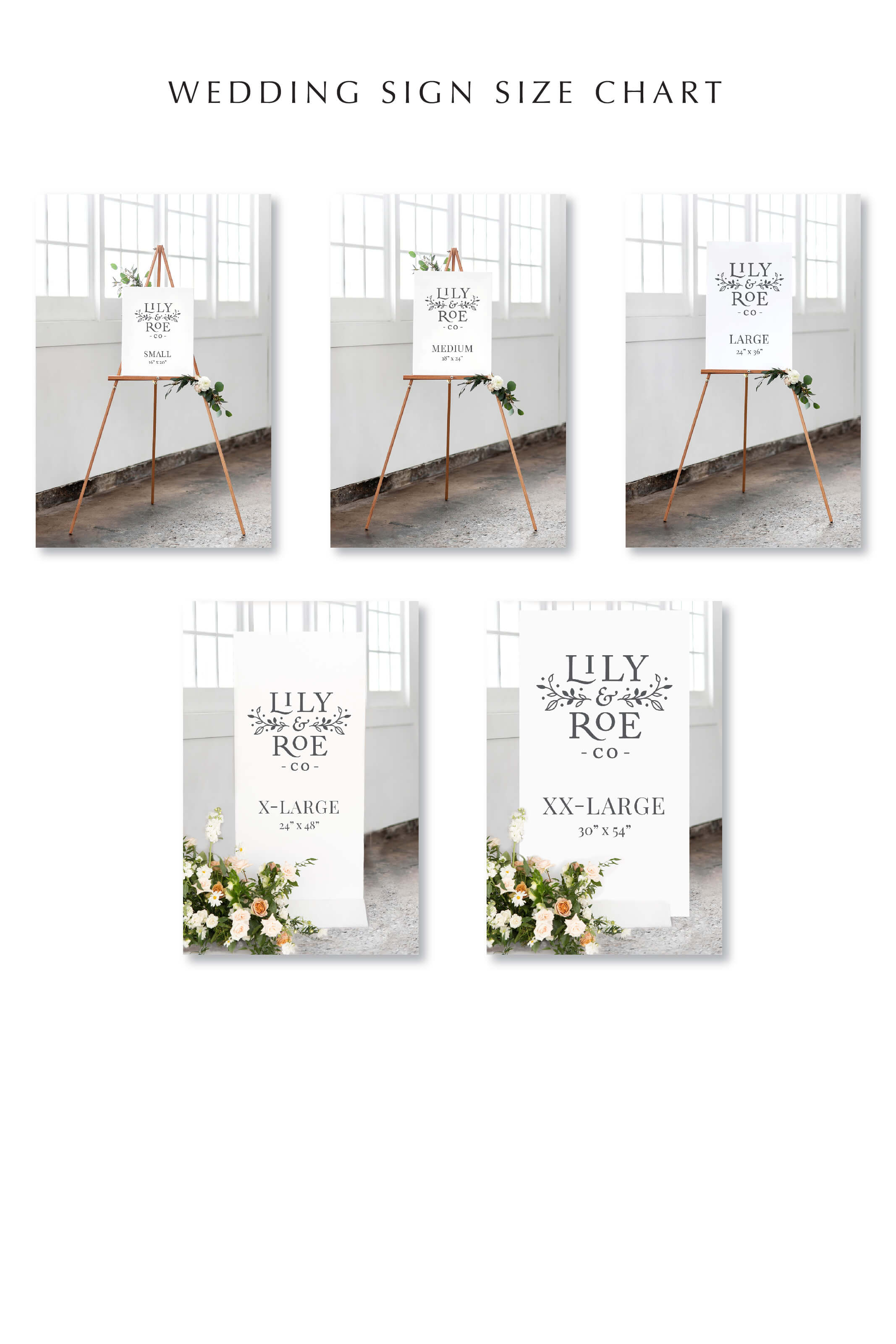The image depicts a wedding sign size chart showcasing five different sign sizes available from the Lilly and Row Company. The signs are displayed in five distinct photos arranged in a grid. At the top of the chart are three vertical rectangles, each displaying small, medium, and large signs, respectively, mounted on a wooden easel. These signs feature a Lilly and Row Company signature at the top, white flowers with green leaves adorning the corners, and the corresponding size labeled below. The bottom row consists of two vertical rectangles featuring the extra-large and double extra-large signs. These larger signs rest on the ground, propped against a wall, also embellished with white flowers in the bottom left corner. The background includes a white wall with four windows halfway up, allowing bright light to filter through, enhancing the visual appeal of the signs.